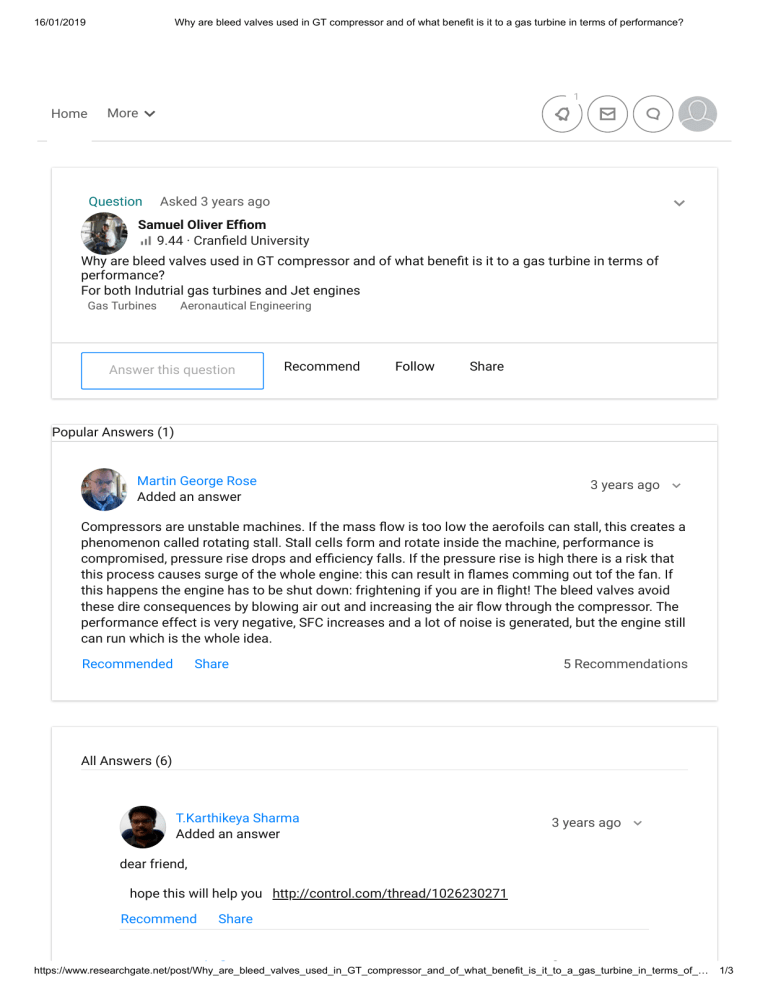The image depicts an online question-and-answer forum interface. At the top of the screen, navigation options such as "Home" and "More" are visible, along with several icons for notifications, messaging, discussions, and user profile. The date at the top reads January 16th, 2019.

The main focus is a question posted by a user, asking: "Why are bleed valves used in GT compressors, and of what benefit is it to a gas turbine in terms of performance?" Below this question are multiple answers in separate rectangles.

The top answer is by Samuel Oliver, FEM, who repeats the initial question for context: "Why are bleed valves used in GT compressors, and of what benefit is it to a gas turbine in terms of performance?" Samuel mentions that this applies to both industrial gas turbines and jet engines.

Directly below, the platform provides options for users to answer, recommend, follow, or share the discussion. Martin George Rose contributes a detailed response, which spans an entire paragraph. His answer, marked as popular, has garnered five recommendations and was posted three years ago.

Further down, T. Karkataya Sharma offers another answer, beginning with "Dear friend, hope this will help you," and includes a hyperlink for additional information. Users can see that the thread displays a total of six answers, with an option to view all responses.